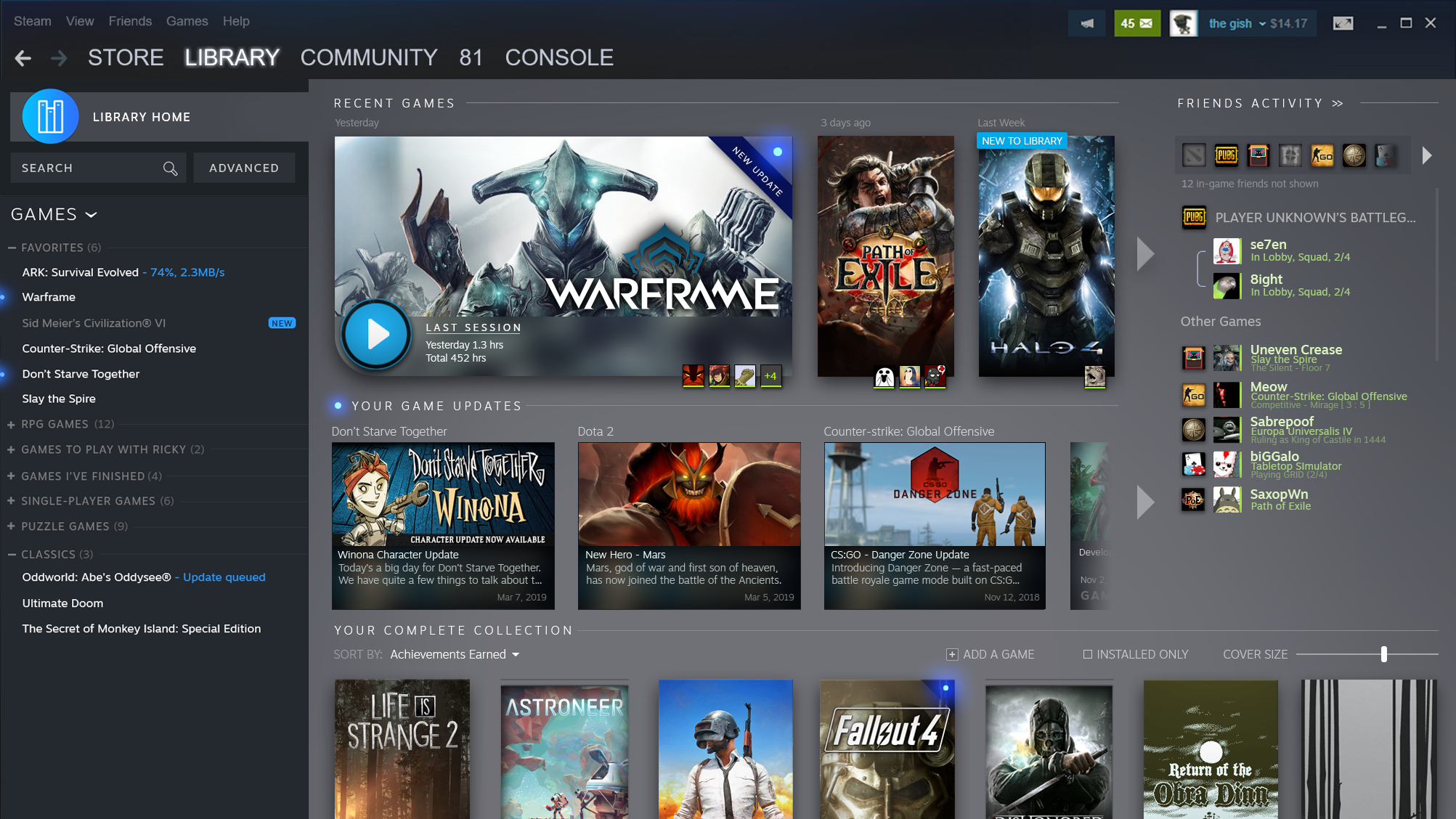The image showcases the Steam store interface on a Windows computer, as indicated by the familiar Windows UI elements in the upper right corner. To the immediate left of these elements, the Steam interface displays the user's profile, showing a balance of $14.17. Next to this is an icon with a number 45 and an envelope, likely indicating notifications or messages, followed by a bullhorn symbol.

On the far left, the top menu bar includes options like "Steam," "View," "Friends," "Games," and "Help." Beneath this menu bar are further navigation tabs: "Store," "Library," "Community (81 notifications)," and "Console." The interface then transitions to the main content area.

In this area, a grid layout displays various game tiles. Prominent titles include "Warframe" on the left, flanked by "Path of Exile" and "Halo 4." Further right, a section labeled "Friends Activity" appears, followed by details about friends currently playing games. It mentions that 12 in-game friends are not shown but highlights "PUBG" with two active players along with other unspecified games being played by friends.

Along the left-hand side, there is a vertical list of the user's owned games against a dark blue background with white text. Notable titles in this list include "ARK: Survival Evolved," "Warframe," "Sid Meier's Civilization," "Counter-Strike: Global Offensive," and "Don't Starve Together."

Overall, the screen is primarily set against a gray background, providing a visually organized and user-friendly interface.